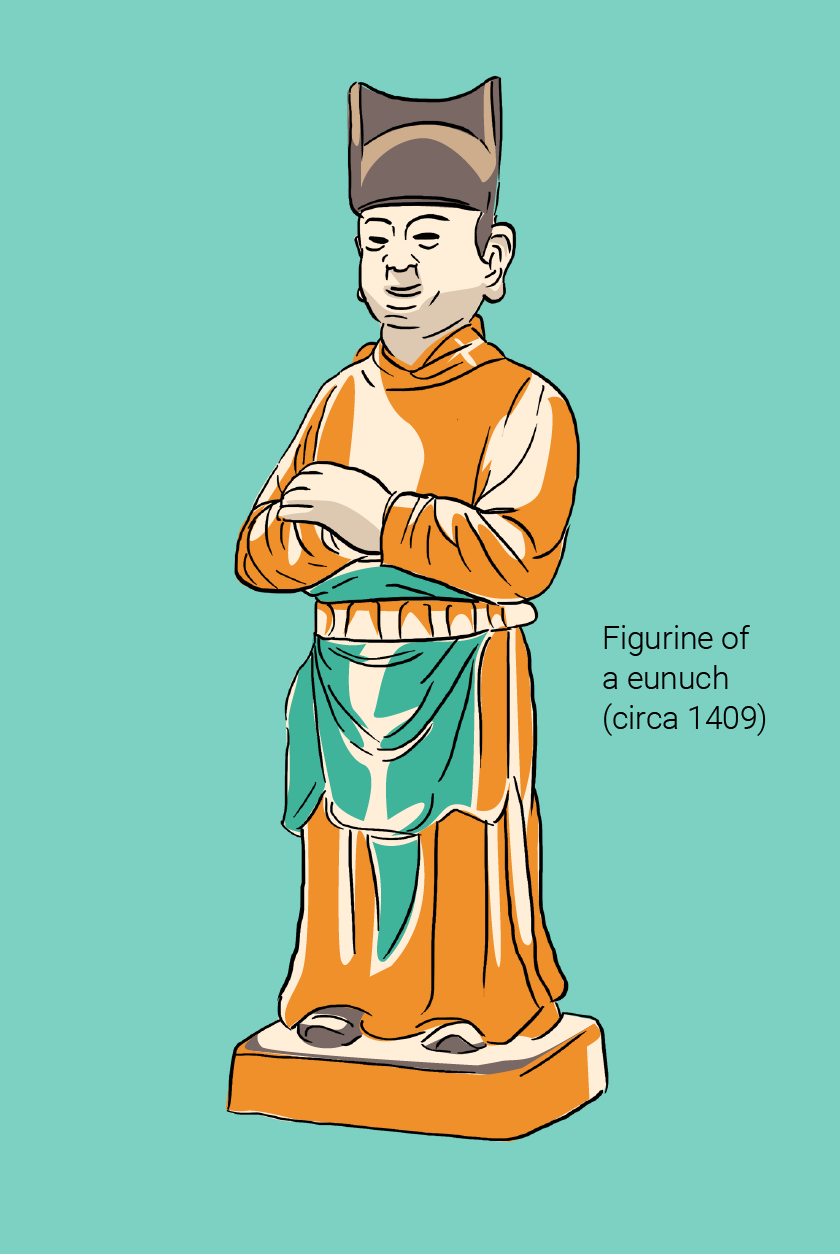The image is a cartoonish drawing of a detailed figurine or sculpture with a distinct Asian, likely Buddhist, style. The figure is depicted wearing an orange robe with white reflective elements and a blue towel-like garment wrapped around his waist, secured with an orange belt featuring white stripes. He has big ears, no facial hair, and wears a gray, curved top hat. His sandals are gray, and he stands on a rectangular block or pedestal. His hands are folded across his chest, and his robe covers him from head to toe. Black lettering on the right-hand side identifies the figure as a eunuch, circa 1409. The entire scene is set against a turquoise blue background, with the figurine drawn in bright colors and outlined in black lines.